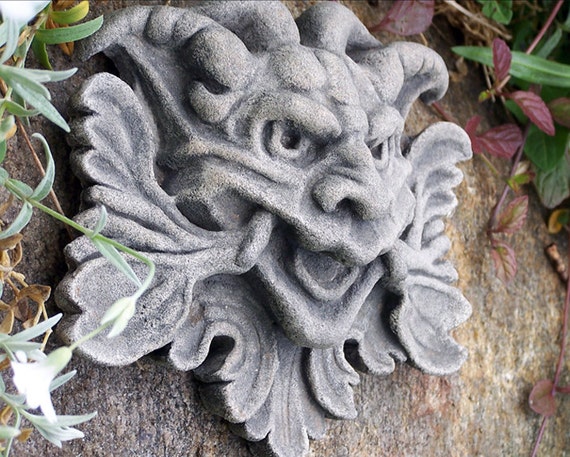This photograph showcases a detailed stone garden ornament depicting a demonic or gargoyle-like head, prominently mounted on the side of a large boulder. The boulder, composed of brown and gray hues, is partially enveloped by an assortment of greenery, including some maroon-colored plants. The stone artwork features a fearsome visage with a wide, open-mouthed grin displaying pronounced teeth and intense eyes. Notably, the creature has four horns emerging from its forehead area, and its neck is adorned with leaf motifs. Surrounding the sculpture, there are white flowers on one side and maroonish-purple leaves on the other, adding to the garden scene's rich texture.